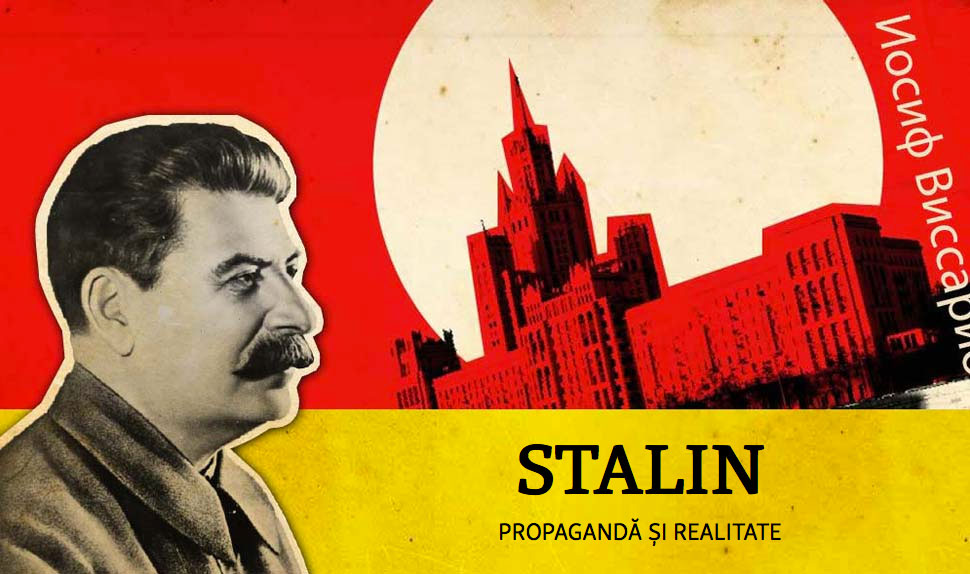The image is a vintage propaganda poster featuring Joseph Stalin. The top two-thirds of the poster consists of a red background with the Kremlin prominently displayed. Behind the Kremlin, a large, perfectly round white circle represents the moon. To the right of the moon, there is some text written in Russian. Covering the bottom third of the poster is a yellow banner. On this banner, the word "Stalin" is bolded in black, followed by the words "Propaganda CSI Realitate." Overlaying the left side, bridging both the yellow banner and the red background, is a black-and-white profile portrait of Joseph Stalin. Stalin is depicted with dark hair slicked back, a bushy mustache, a long nose, dark eyebrows, and dark eyes, dressed in a dark jacketed suit. The poster combines elements of Soviet symbolism and propaganda, with text in multiple languages, potentially from a website or digital source.